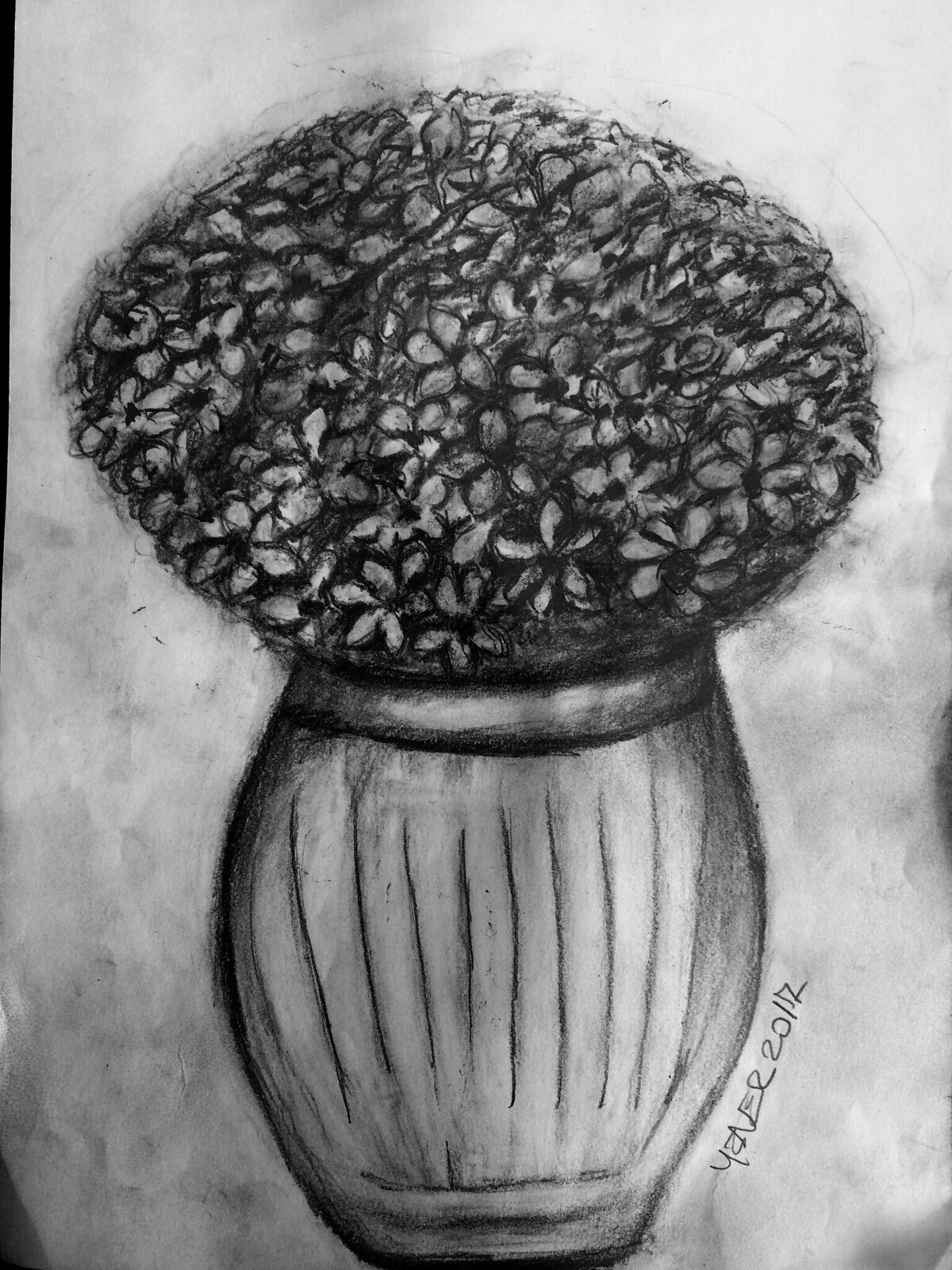A black-and-white drawing features an intricately detailed vase brimming with an abundance of flowers, creating the impression of a flourishing bush. The vase, which appears to be artificial, has a cylindrical shape adorned with vertical black lines reminiscent of a barrel, accompanied by two horizontal lines encircling the top and bottom. The shading and texture of the drawing exhibit a chiaroscuro technique, emphasizing the contrast between light and dark. In the lower corner, the artwork is signed with what looks like "Jaeger 2012," though the signature is somewhat difficult to decipher.